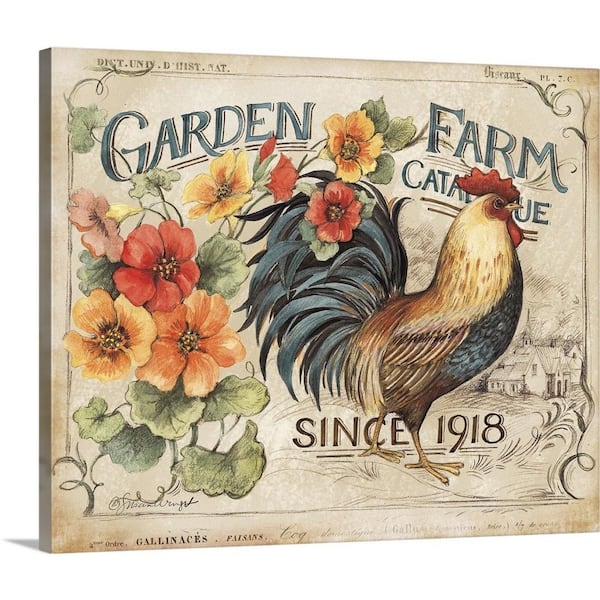The image showcases a vertically standing, square-shaped garden sign with a light gray background. The design features an array of detailed elements. On the bottom left, the text reads "G-A-L-L-I-N, aces," accompanied by a small black cursive signature just above it. The design incorporates green leaves, a curly brown vine on the left, and an assortment of colorful flowers: an orange, yellow, and red flower followed by more green leaves, a pinkish-brown flower, another yellow flower, three red flowers, another yellow flower, and three green leaves.

Prominently featured is a rooster with a black and light brown body, a black tail, and a red comb. The sign partially reads "Garden Farm, C-A-T-A," with the remaining letters obscured, and "U-E." Below, the text "since 1918" is written in brown.